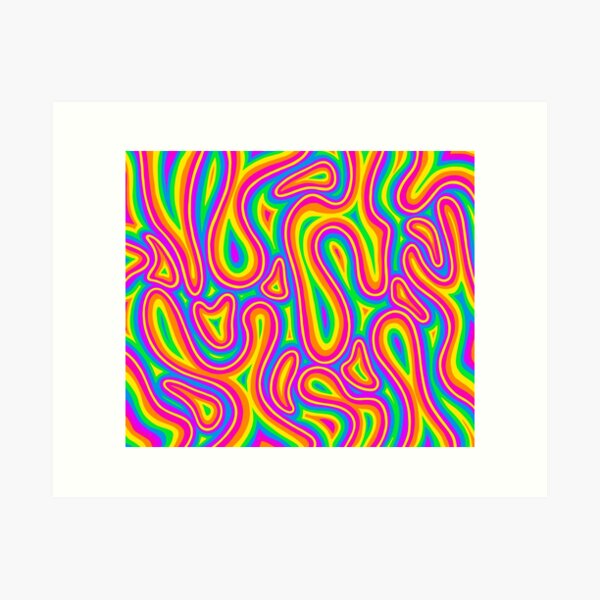The image is a rectangular piece filled with a vibrant, neon-colored, squiggly design that almost appears to move due to its vivid hues and dynamic patterns. The squiggles intertwine in colors of blue, green, yellow, orange, red, pink, and purple, creating an illusionary, almost 80s funk or disco-inspired aesthetic. It's set within a white border, which is surrounded by a larger gray square background. The colors are tightly packed, resembling a mass of worms or abstract shapes in various forms such as teardrops and circles. Despite its whimsical and chaotic appearance, the image, captured on a matte surface, lacks a clear intent or specific subject, making it feel energetic yet somewhat disorienting.